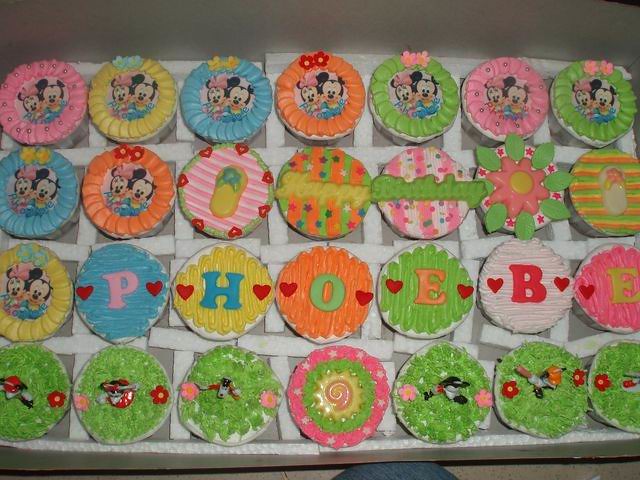This is a vibrant color photo of a neatly arranged assortment of 28 cupcakes, set on a blue and white tablecloth. The cupcakes are organized into four rows and seven columns. The top row features cupcakes with adorable Mickey and Minnie Mouse decorations in the center, surrounded by pink, yellow, blue, orange, and green icing rings. The second row contains colorful cupcakes, two of which prominently display the words "Happy Birthday." In the third row, the name "Phoebe" is spelled out in different colored letters, with each cupcake bearing one letter and adorned with little red hearts on either side of the letter. The lower row continues to showcase a variety of brightly decorated cupcakes with green icing and other colorful decorations. The cupcakes are arranged in a large pan, creating a visually appealing and festive display suitable for a birthday celebration.